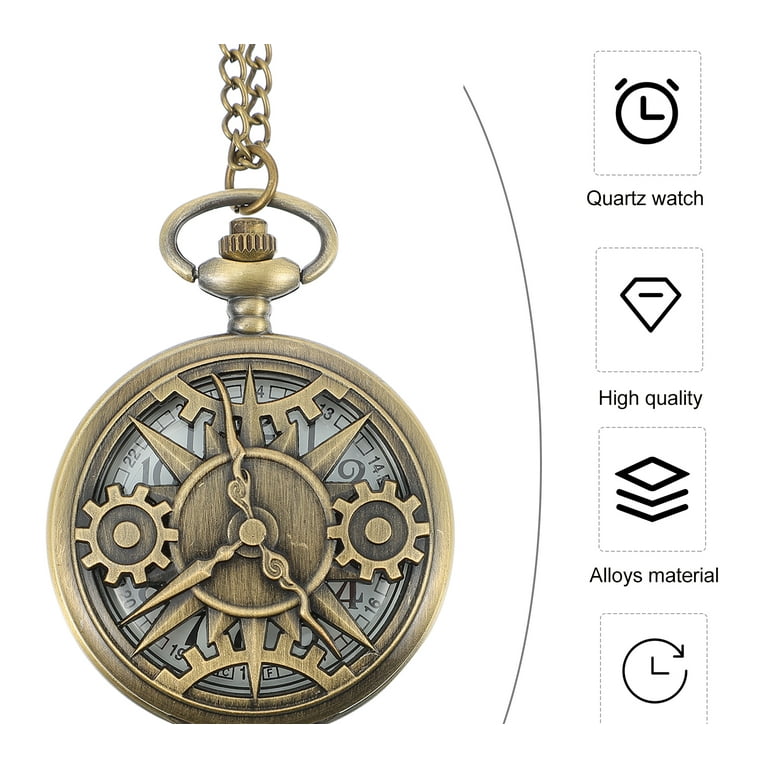This image is an advertisement for a brass or gold-colored pocket watch with a steampunk design. The watch is suspended by a chain attached to a ring above the winding stem. The front cover features an intricate design with ornamental gears on the left and right sides and larger semi-circle gears on the top and bottom. These gears are decorative and do not move. The cover has cut-out sections that reveal the true white dial face of the watch beneath, which displays black and gray numbers and three curvy hands for the hour, minute, and second. On the right side of the image, there are four labeled icons providing information about the watch. The top icon is a clock face labeled "Quartz Watch," the second icon is a diamond labeled "High Quality," the third icon shows stacked sheets labeled "Alloys Material," and the bottom icon is partially cut off but depicts a clock with a circular arrow indicating clockwise rotation. The entire advertisement is set against a pristine white background, with the chain clipped at the edge of the image.